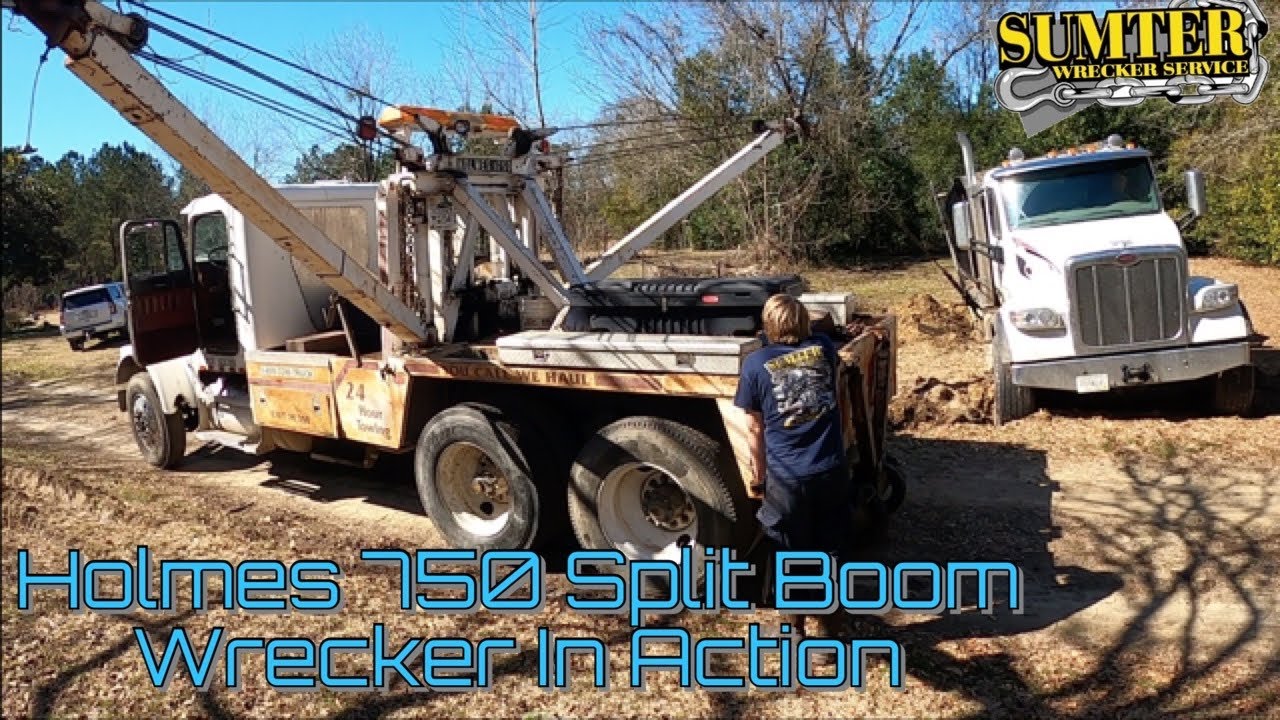This outdoor photograph, taken in landscape mode, captures a vibrant scene involving a tow truck from the Sumter Wrecker Service. Prominently displayed on the top right corner is the company's logo, encircled by chain links symbolizing their towing service. Central to the image is a white tow truck with the driver's side door ajar, revealing its operational state. A man in a blue graphic t-shirt and matching cargo pants stands at the rear end of the truck, actively engaged in loading or handling equipment, illustrating the truck in action as noted by the blue caption at the bottom: "HOLMES 750 SPLIT BOOM WRECKER IN ACTION." To the right, a complementary work truck with a crane extends into view, bearing "24-hour towing" on its rusted side, further highlighting the round-the-clock service. In the backdrop, a silver SUV is partially visible against a wooded landscape, adding depth to the dirt road setting, which basks in the clear sunlight.